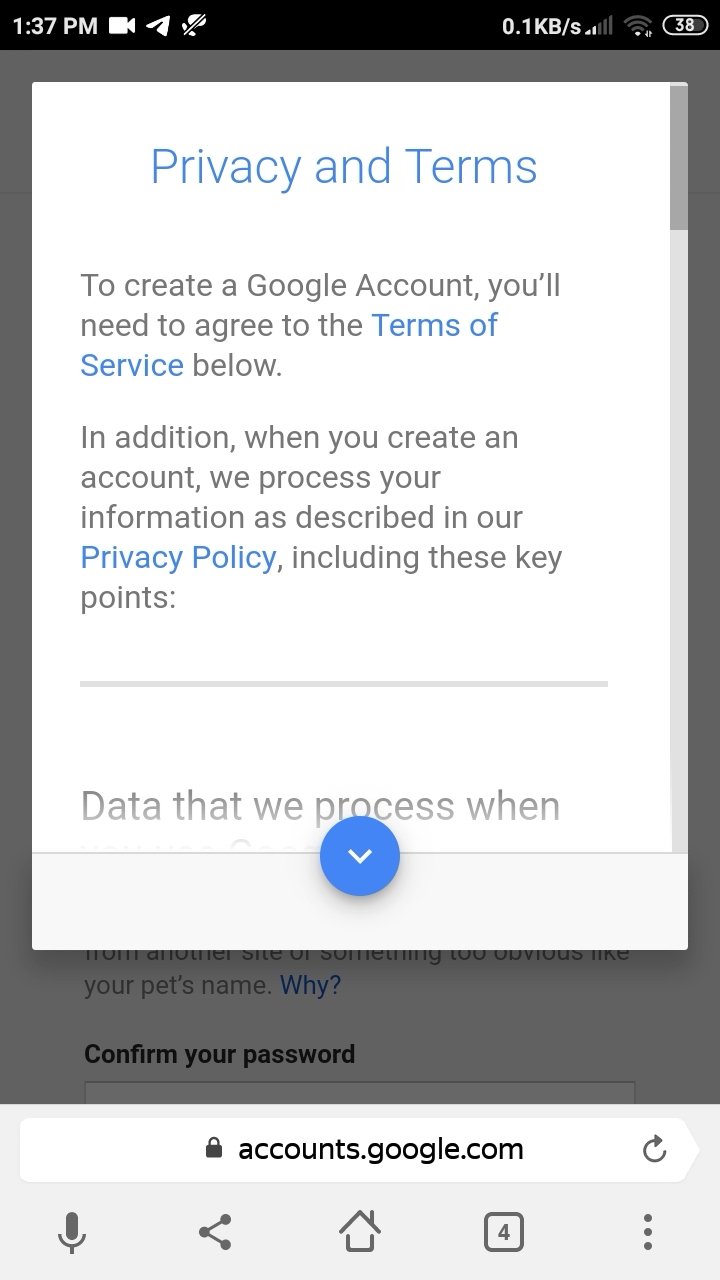This is a detailed screenshot from a mobile phone showcasing a Google account creation page. The top of the screen features a black status bar with various white icons and text displaying, from left to right: the time (1:37 PM), recording icon, messaging icon, an unrecognized icon, and on the far right, 0.1 kilobytes, two bars of mobile reception, one bar of Wi-Fi signal, and a battery icon showing 38% charge.

Below this, the screen has a grayish background with faint text and a white pop-up box superimposed. This popup features black and blue text where the essential details are highlighted: 
- "Privacy and Terms" title
- Notification stating, "To create a Google account, you will need to agree to the Terms of Service below. In addition, when you create an account, we'll process your information as described in our privacy policy, including these key points."

A horizontal line divides this section from a subsequent text beginning with "Data that we process when...", indicating further details can be revealed by scrolling down.

Lower in the window, a hint of blue text reads, "your pet's name," followed by "Confirm your password," suggesting input for password confirmation and advice against using easily guessable passwords like pet names.

The footer of the screen shows the URL "accounts.google.com" with a padlock icon ensuring a secure connection, plus a reload icon on the right for refreshing the page.

At the very bottom, navigation icons are visible, including record, share, home, tab management (with four squares), and a menu option represented by three vertical dots, located at the lower right corner.